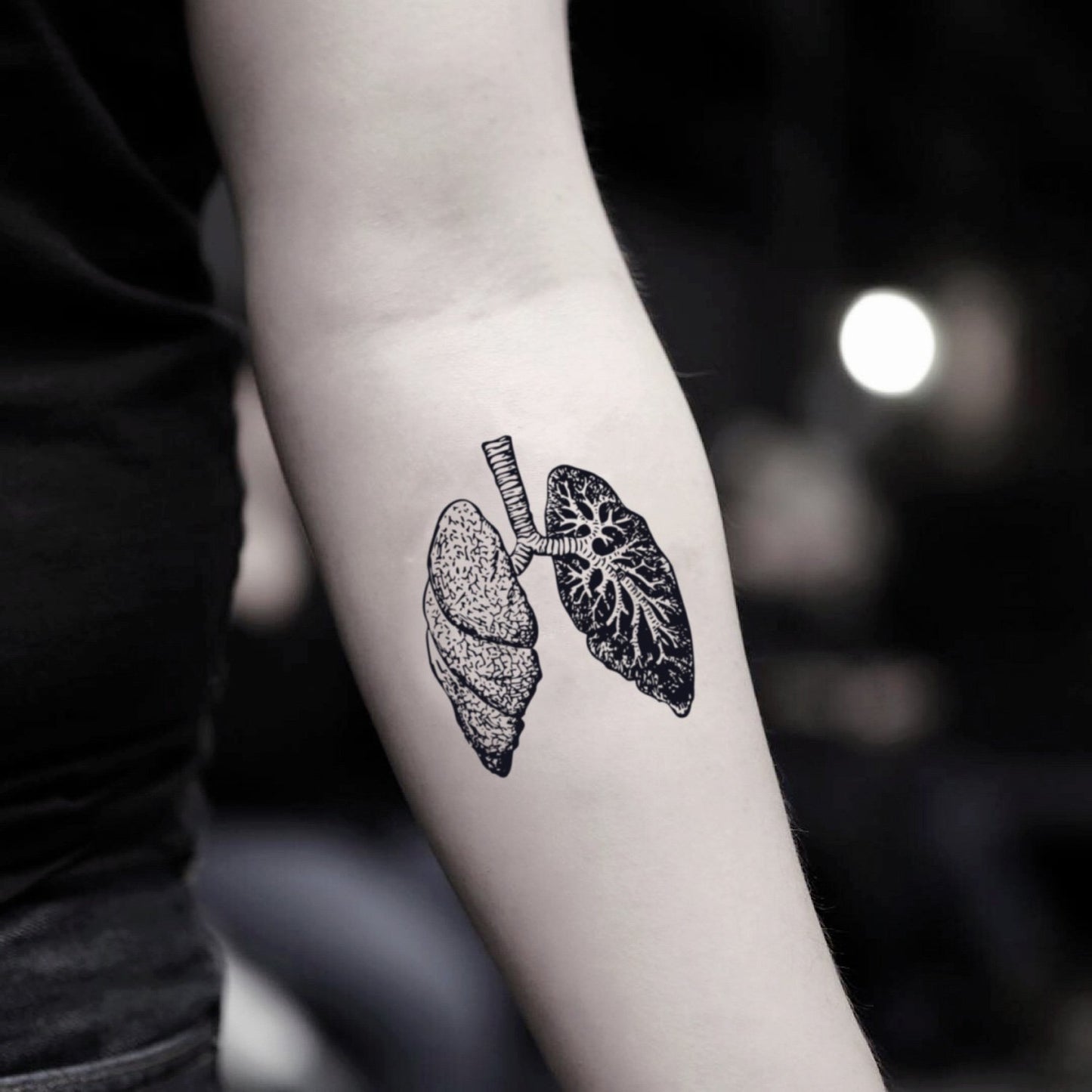This is a photograph, almost monochromatic in tone, depicting a portion of a person's forearm adorned with an intricately detailed tattoo. The arm, positioned diagonally from the top left to the bottom right, is cropped above the wrist and below the shoulder. The tattoo, which is a black line art illustration of human lungs, is located near the crease of the elbow. The left lung displays its outer surface, marked with speckles, while the right lung reveals a more detailed inner framework, including veins that look like little roots. Alongside the arm, a small section of the person’s body is visible, clad in a black t-shirt and jeans. The background is blurred and dark, with a faint round-shaped white light source visible, contributing to the realistic yet representational style of the image.